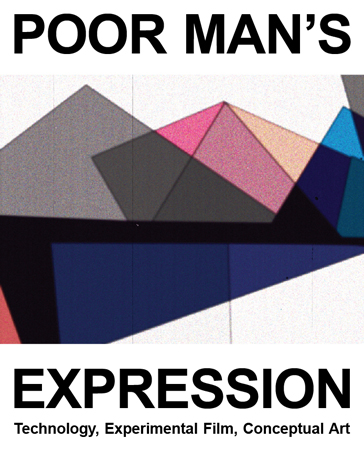This image serves as the cover for a publication, prominently featuring both its title and subtitle. At the top, the title "Poor Manz" is displayed, while the bottom showcases the descriptors: "Expression, Technology, Experimental Film, Conceptual Art."

Dominating the center of the cover is an intricate array of three-dimensional shapes, each unique in form yet collectively exuding a diamond-like appearance. These shapes are a medley of vibrant and varied colors, including shades of blue, dark blue, pink, light pink, light orange, dark gray, and light gray. Their structure resembles pyramids composed of interconnected triangular facets, creating a visually stimulating and somewhat basic geometric pattern. The overall effect is a complex, kaleidoscopic mosaic that entices the viewer with its rich diversity and conceptual depth.